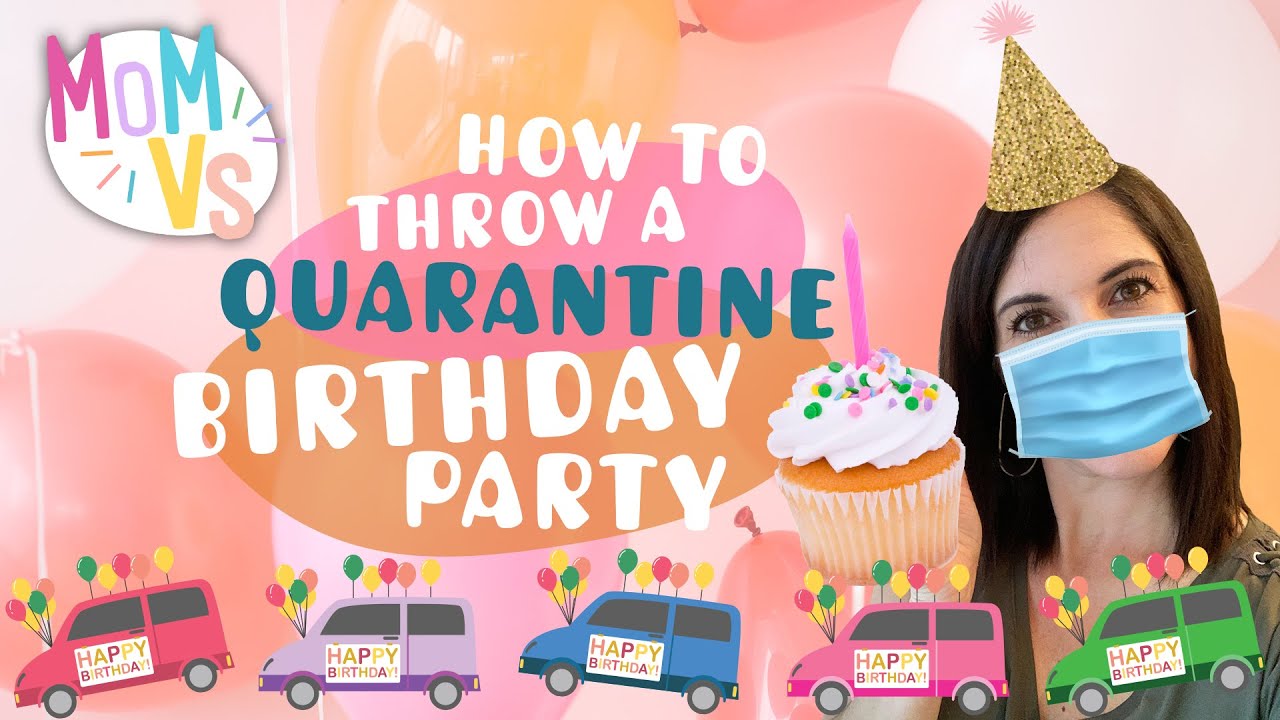This landscape-oriented image, likely a professionally designed poster or a still frame from a YouTube video, is vibrant and celebratory. The focal point features two overlapping ovals, one pink and one orange, displaying the title "How to Throw a Quarantine Birthday Party" in a playful combination of white and blue text. 

In the upper left corner, the logo "Mom vs." or "vs." is prominently displayed within a circle. A whimsical caravan of cartoon cars, each adorned with colorful balloons and the message "Happy Birthday," lines the bottom of the image. These cars are depicted in a range of colors, including yellow, red, green, pink, orange, and blue, all moving toward the left.

Dominating the right side of the poster, a photograph of a woman adds a personal touch. She wears a blue surgical mask and a glittery gold cone birthday hat trimmed with pink feathers. Holding a cupcake with white frosting and a pink candle, she is surrounded by a festive array of balloons in shades of black, white, gray, blue, pink, orange, green, and various other shades of pink. Her brown hair peeks out from under the hat, complementing the overall celebratory atmosphere of the image.